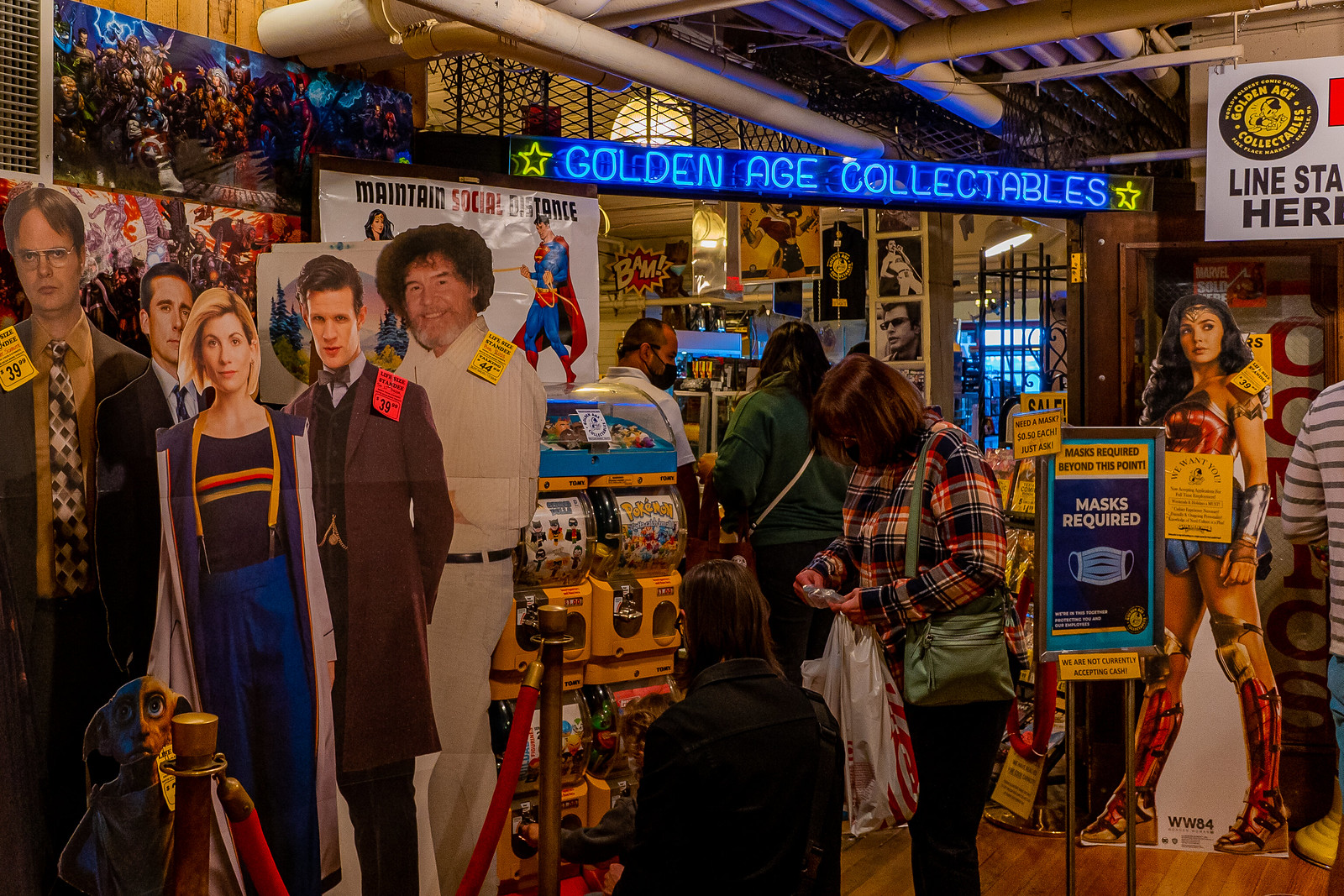The photograph captures the interior of a highly cluttered room, brimming with various objects and paraphernalia reminiscent of a vibrant pop culture store. On the left side of the image, several cardboard cutouts stand tall, featuring popular figures such as Doctor Who and characters from The Office. Behind these cutouts, small gold and blue toy dispensers are partially visible. Toward the right side, another cardboard cutout of Wonder Woman catches the eye. Adjacent to Wonder Woman on her left stands a sign with a blue background, clearly stating "Masks Required" in white text.

Above, an eye-catching neon sign glows brightly, reading "Golden Age Collectibles" framed by neon stars on both sides. The room is bustling with activity, as several people can be seen within the space. In the center of the image, a woman and a child are present, both facing away from the camera. The distant walls, though obscured by the overwhelming amount of superhero and media-themed merchandise, contribute to the overall sense of organized chaos. The ceiling is lined with white, exposed pipes, adding to the industrial feel of the room.